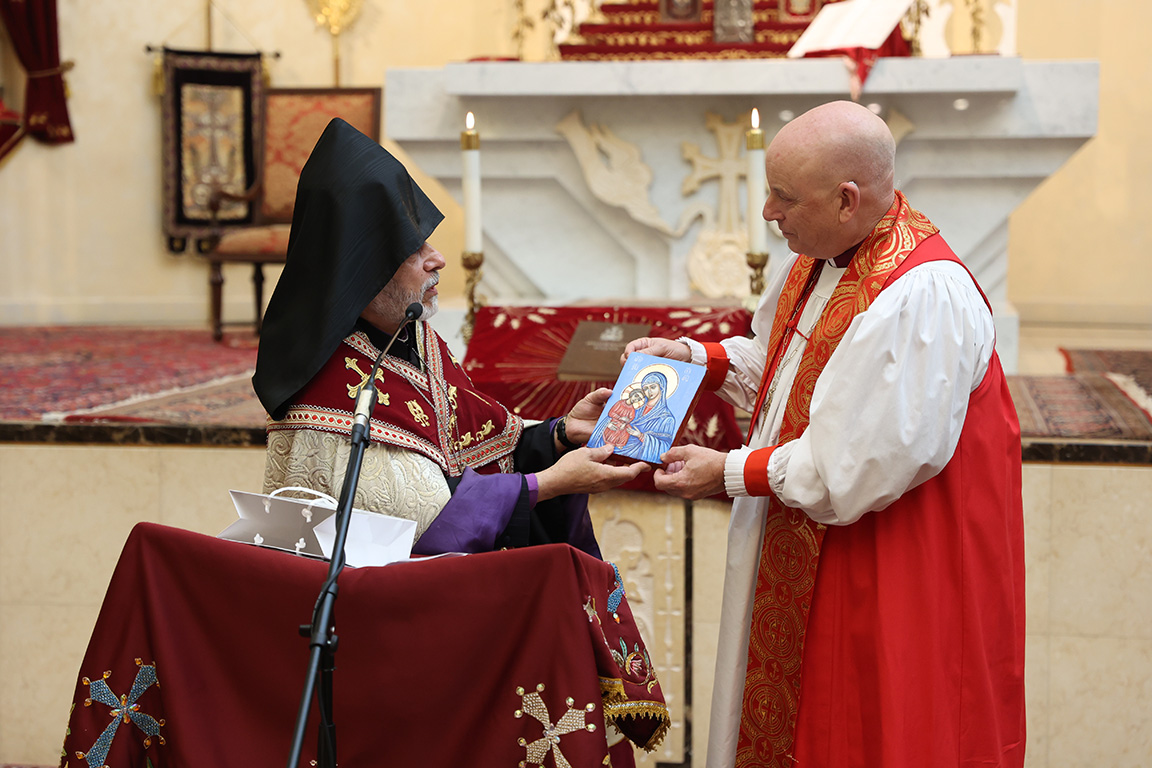In this detailed photograph, taken inside a Catholic church, two older men, possibly priests or bishops, are depicted standing at the altar in front of a stage adorned with decorations, a white altar, and lit candles. The man on the left, wearing a black hat or hood, is dressed in a white robe with purple accents and a burgundy shawl draped around his shoulders. He has a microphone positioned near his mouth and is resting his hands on a podium covered with a burgundy cloth featuring crosses. This man appears to be handing or receiving a small religious picture or card, likely depicting the Virgin Mary and Jesus, from the man on the right. The man on the right, who is bald, is attired in a white garment with a red vest and a matching red and gold scarf. Both men are facing each other, engaged in what seems to be a ceremonial exchange of gifts within the church’s sacred setting.